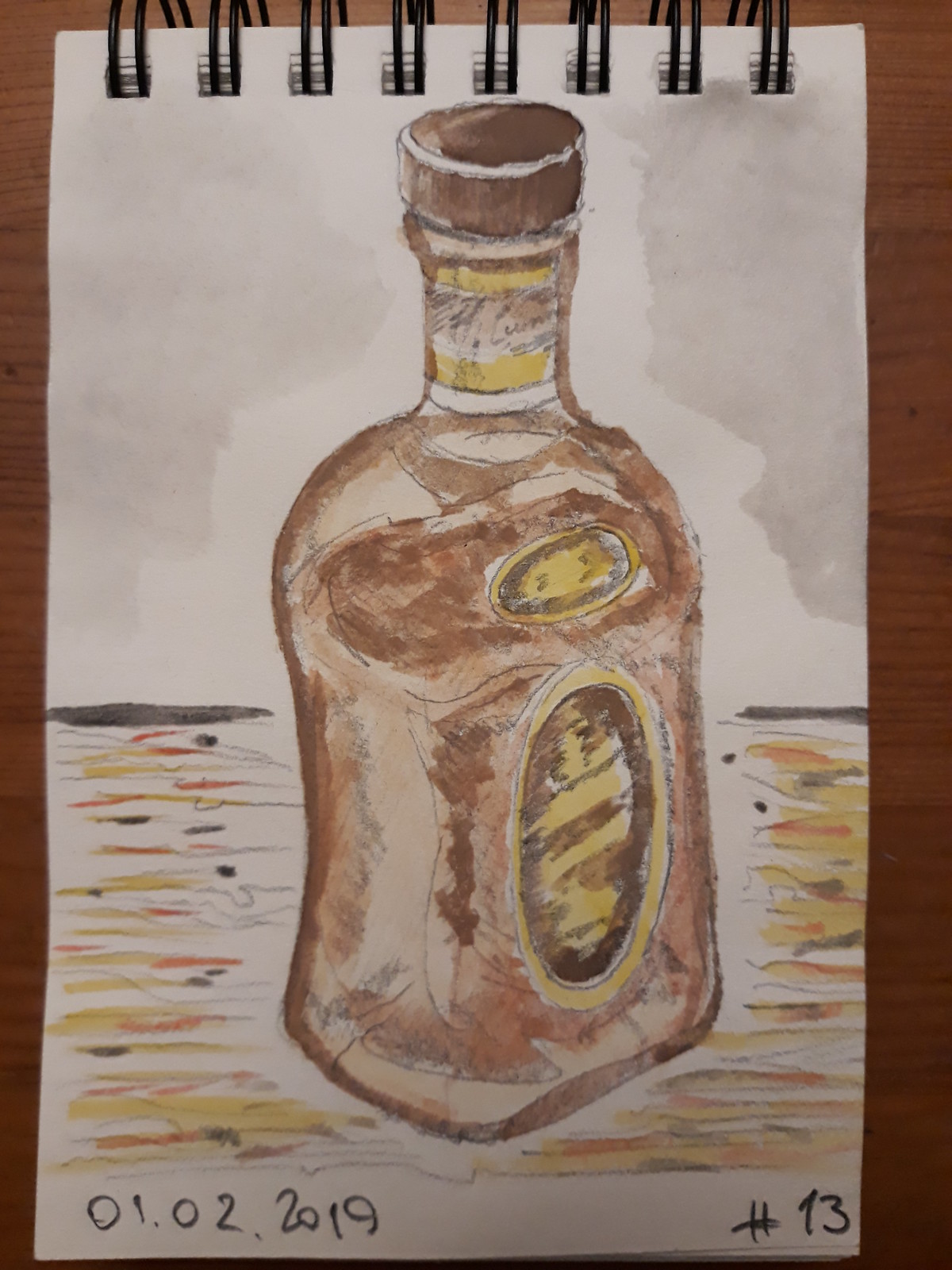This image showcases a detailed sketch laid on a brown table. The sketch is on a white page within a spiral notebook, with the black spiral prominently visible at the top. Central to the sketch is a detailed depiction of a bottle, which appears to be a liquor bottle. The bottle features a brown cap and a yellow section around its neck. The lower part of the bottle is shaded in brown, adding depth to the drawing. Towards the middle of the bottle, there is a small yellow oval, complemented by a larger oval shape in the front, which is brown with a yellow center. The background behind the top of the bottle is subtly shaded in gray, contrasting with the predominantly yellow foreground that features hints of red and black dots. In the bottom left corner of the notebook page, the date "01.02.2019" is inscribed, while "number 13" is noted in the bottom right corner.